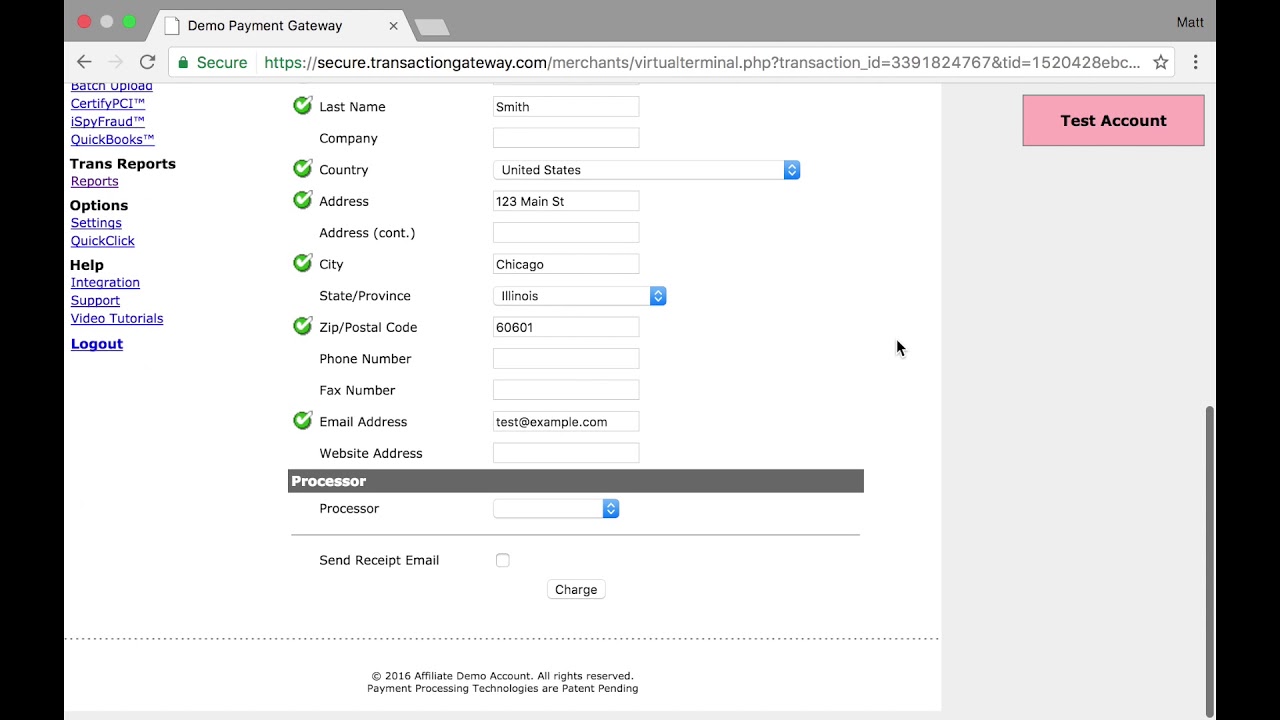The image features a web interface with a secure and detailed layout for a payment processing gateway.

At the top of the interface, the tab reads "Demo Payment Gateway," and the address bar displays "SecureTransactionGateway.com."

The left sidebar contains a series of navigation links in blue, namely: Batch Upload, Certified PCI, Spy Fraud, QuickBooks, Trans Reports, Options, Settings, Quick Click, Help, Integration, Support, Video Tutorials, and Log Out.

The central portion of the interface contains several form fields for inputting personal and business information. These fields are labeled: Last Name, Company, Country (pre-filled with "United States"), Address (with "123 Main Street" entered), Address Continued, City (entered as "Chicago"), State/Province (entered as "Illinois"), ZIP/Postal Code (entered as "60601"), Phone Number, Fax Number, Email Address (entered as "test@example.com"), and Website Address.

Below these form fields is a narrow black band with white text that reads "Processor." Further down, there are additional options: Processor, Send Receipt Email, and a black button labeled "Charge."

At the bottom of the interface, a footer notes "Copyright 2016, Affiliate Demo Account, All rights reserved. Payment processing technologies are patent pending."

Additionally, in the upper left corner, a red button labeled "Test Account" is prominently displayed, indicating the user is in a test environment.